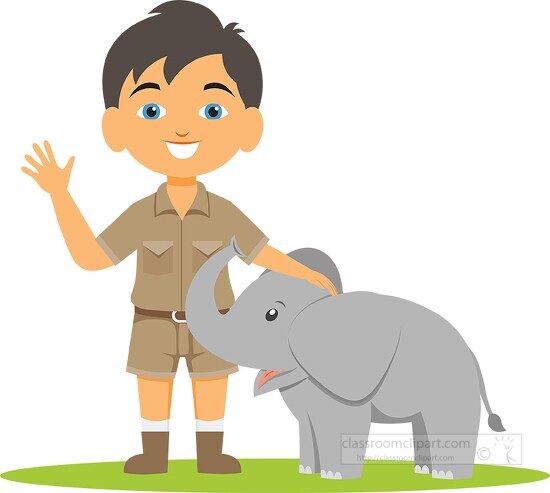This is a computer-generated illustration featuring a young Caucasian boy with dark hair and blue eyes. He is dressed in a short-sleeved safari shirt, complete with two chest pockets, a brown belt with a silver buckle, matching brown shorts, brown shoes, and white socks. The boy is portrayed standing on a green patch of grass, with his hand gently resting on the top of a baby elephant beside him. The elephant, which reaches up to the boy's waist, has its trunk playfully curled towards the boy's right arm and an open mouth revealing a pink tongue. In the bottom right corner of the illustration is a rectangular logo of "http://classroomclipart.com" with a copyright symbol. The logo also includes a stick figure with arms outstretched, one leg kicked up, and lines emanating from its head like sunbeams, indicating excitement or joy.